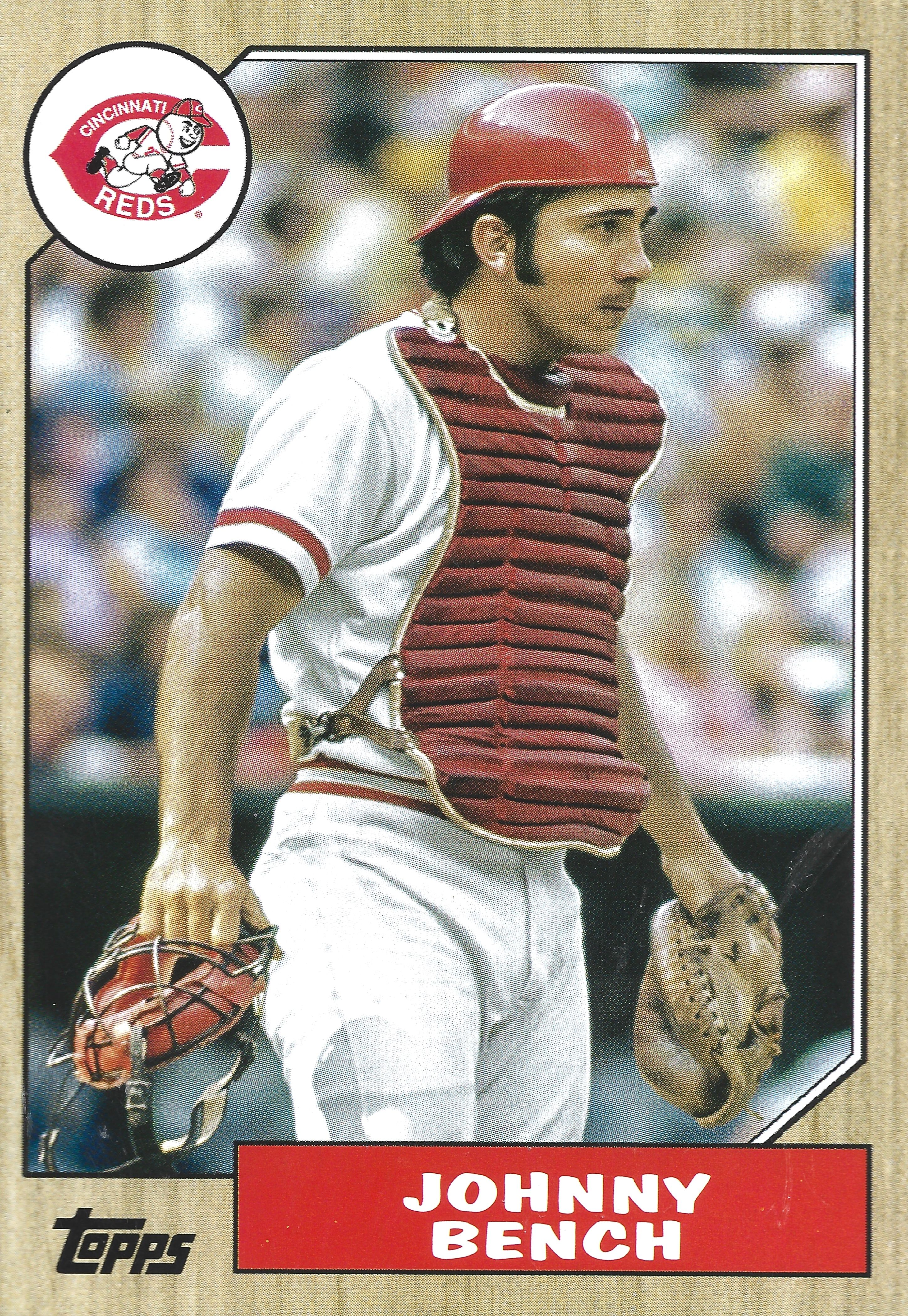This photograph captures a young Johnny Bench during his time as a catcher for the Cincinnati Reds. Set within a wooden border, the image prominently features Bench standing and facing to the right, decked out in his catcher gear. He sports a white uniform with red stripes on the sleeves and a black batting helmet worn backwards, indicative of his position behind the plate. His protective chest guard is clearly visible, and he holds his catcher's mask in his right hand while his mitt is on his left. Bench's long, dark sideburns and dark hair are noticeable under the helmet. In the background, the blurry outlines of fans fill the stands, adding to the action-packed atmosphere. The card has notable features: at the lower left corner, the word "TOPS" is inscribed, and to the right, "Johnny Bench" is displayed in white text over a red background. Additionally, the upper left corner features the Cincinnati Reds logo with a running baseball player whose head is a baseball, emphasizing Bench's connection to the team.